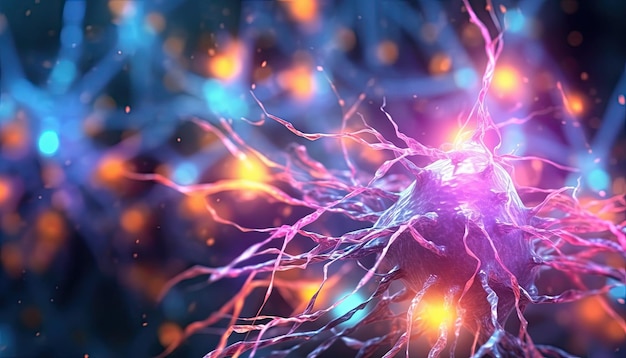The image features a highly abstract composition with a black and blurry dark blue background, speckled with bright orange dots reminiscent of glowing embers or lights, creating a celestial or festive atmosphere. Dominating the center foreground is a smooth, pinkish, circular object that resembles a bald skull. This central object is surrounded by thin, bright white and purple tentacle-like strands that extend outward in various directions, giving the appearance of electrical currents or neural axons and dendrites. On the right side of the image, a structure that looks like illuminated roots or shattered glass adds to the complexity, intertwining with the tentacles from the central form. The overall effect is futuristic, organic, and electric, with both foreground and background elements providing a sense of dynamic, chaotic energy.